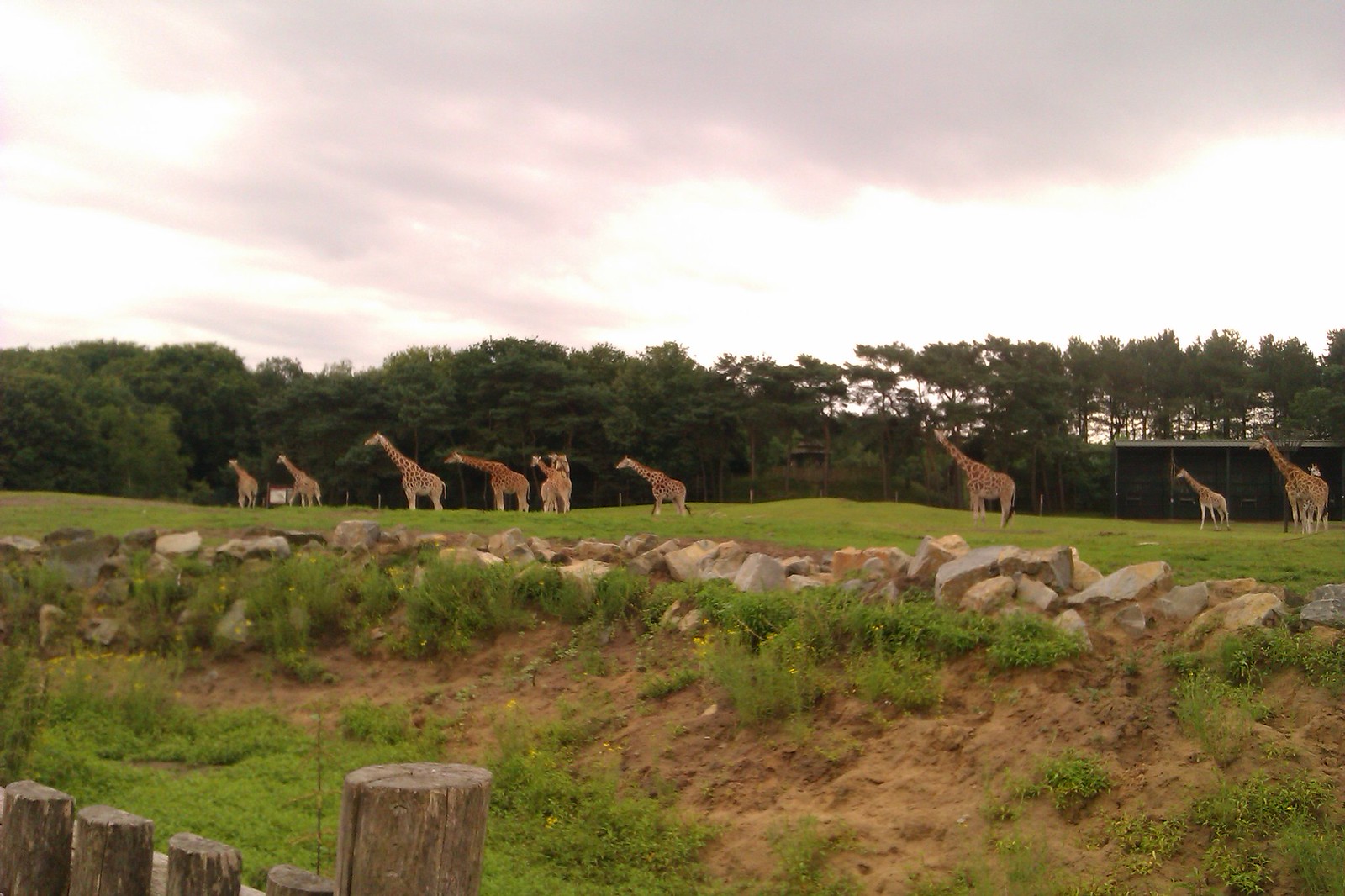In the foreground of this photo, a wooden fence made of vertical posts is visible in the southwest corner, partially framing the scene. Just beyond the fence, there is a muddy embankment lined with large stones, possibly to prevent erosion or to create a boundary. This embankment slopes down to a grassy expanse that stretches across the image. Scattered across this vibrant green field are nine giraffes, their heads and necks all facing towards the left of the image. The giraffes, appearing somewhat small and indistinct, include what looks like a baby or adolescent among them. In the background, near a tree line, there is a structure that appears to be a building that might store farm equipment or feed. This structure is situated to the right-center of the photo, contributing to the sense of a well-maintained area that could be a wildlife sanctuary or preserve. A tall row of trees demarcates the edge of the plain, while the sky above is bright yet overcast with grayish clouds. The scene is serene, with the morning or evening light filtering softly through the clouds.